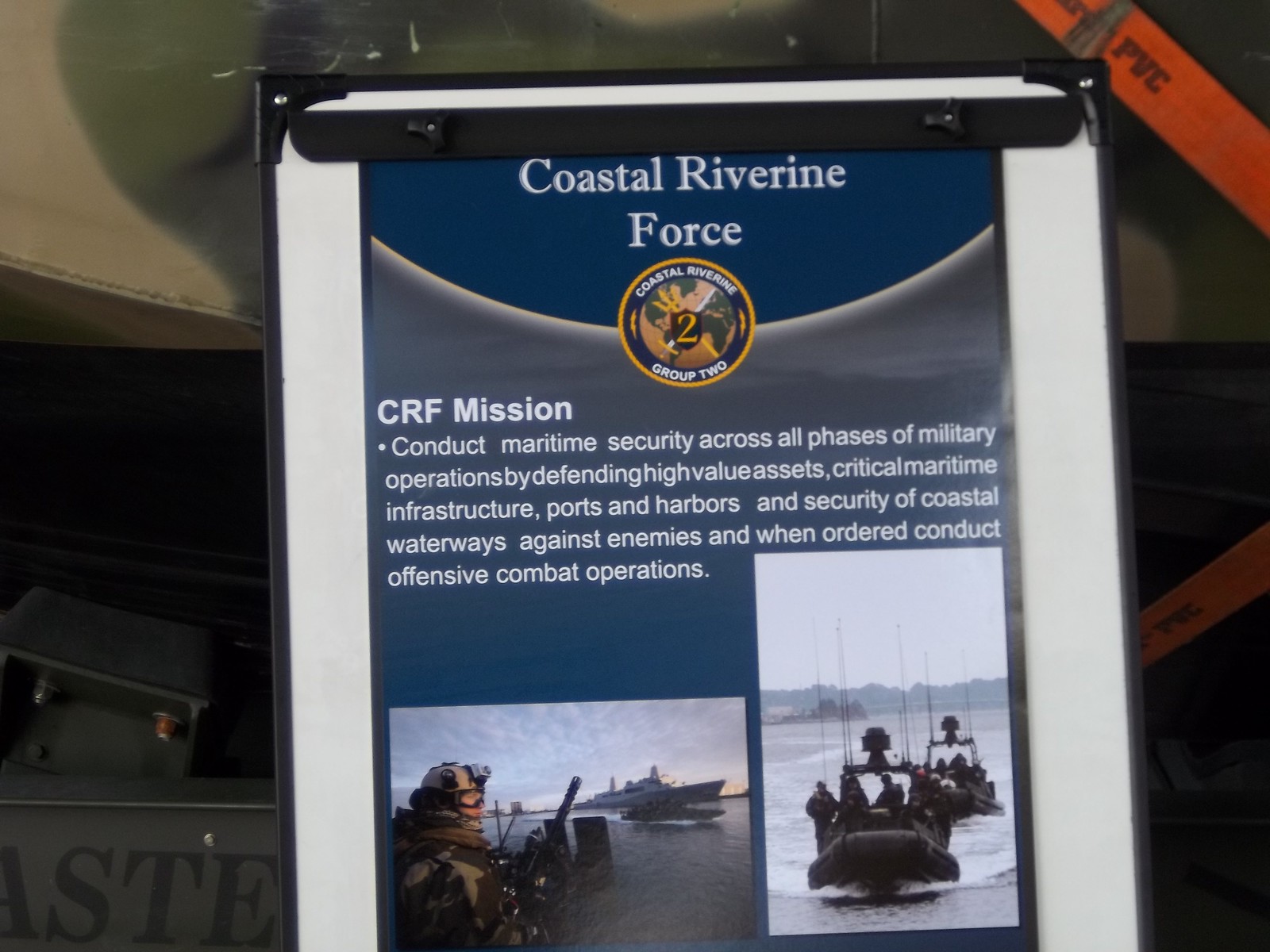The detailed sign is prominently displayed, likely in front of a building or a room. It has white borders and a shiny top surface, with the main background being dark gray. At the top, in a navy blue semicircle with white letters, it reads "Coastal Riverine Force." Below this title, there's a circular badge featuring the Coastal Riverine Group 2 insignia: an outer yellowish-orange circle, an inner blue circle with "Coastal Riverine" at the top and "Group 2" at the bottom, and a gold-colored number 2 in the center.

Underneath this badge, in white text on the dark gray background, the mission statement of the CRF (Coastal Riverine Force) is detailed: "Conduct maritime security across all phases of military operations by defending high-value assets, critical maritime infrastructure, ports and harbors, and security of coastal waterways against enemies, and when ordered, conduct offensive combat operations."

At the bottom of the sign, there's a pair of photographs. The left photo depicts an artillery gunner standing on the deck of an armored ship, aiming out towards the sea, with the ship visible in the background. The right photo shows two pontoon boats on the water, each with several soldiers, against a darkened background with indistinct objects behind them.